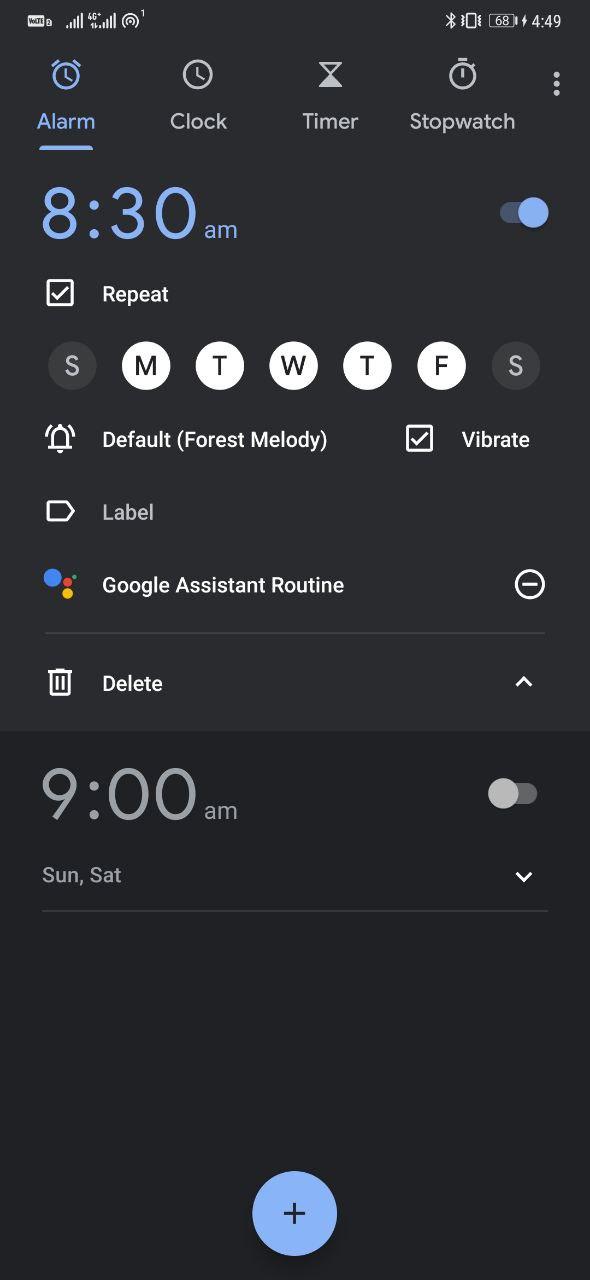This screenshot from a mobile phone displays the settings of a clock app. At the very top, there's a status bar showing various icons: on the left, full mobile signal and Wi-Fi connectivity, along with two unidentified icons. On the right side of the status bar, there are icons for Bluetooth, vibration mode, and a battery icon indicating 68% charge. The time is displayed as 4:49 PM, all in white text against a dark gray, charcoal-like background.

Below this status bar, the clock app’s interface is visible, divided into four tabs: Alarm, Clock, Timer, and Stopwatch. Each tab features an icon above it – an alarm clock for the Alarm tab, a clock face for the Clock tab, an hourglass for the Timer tab, and a stopwatch for the Stopwatch tab. The Alarm tab is selected, highlighted in blue, while the other tabs are in white.

The main content area for the alarm settings shows a large, bold "8:30 AM" in blue font, indicating the set time for the alarm. There’s a toggle button beside this time, which is activated, signifying that the alarm is turned on.